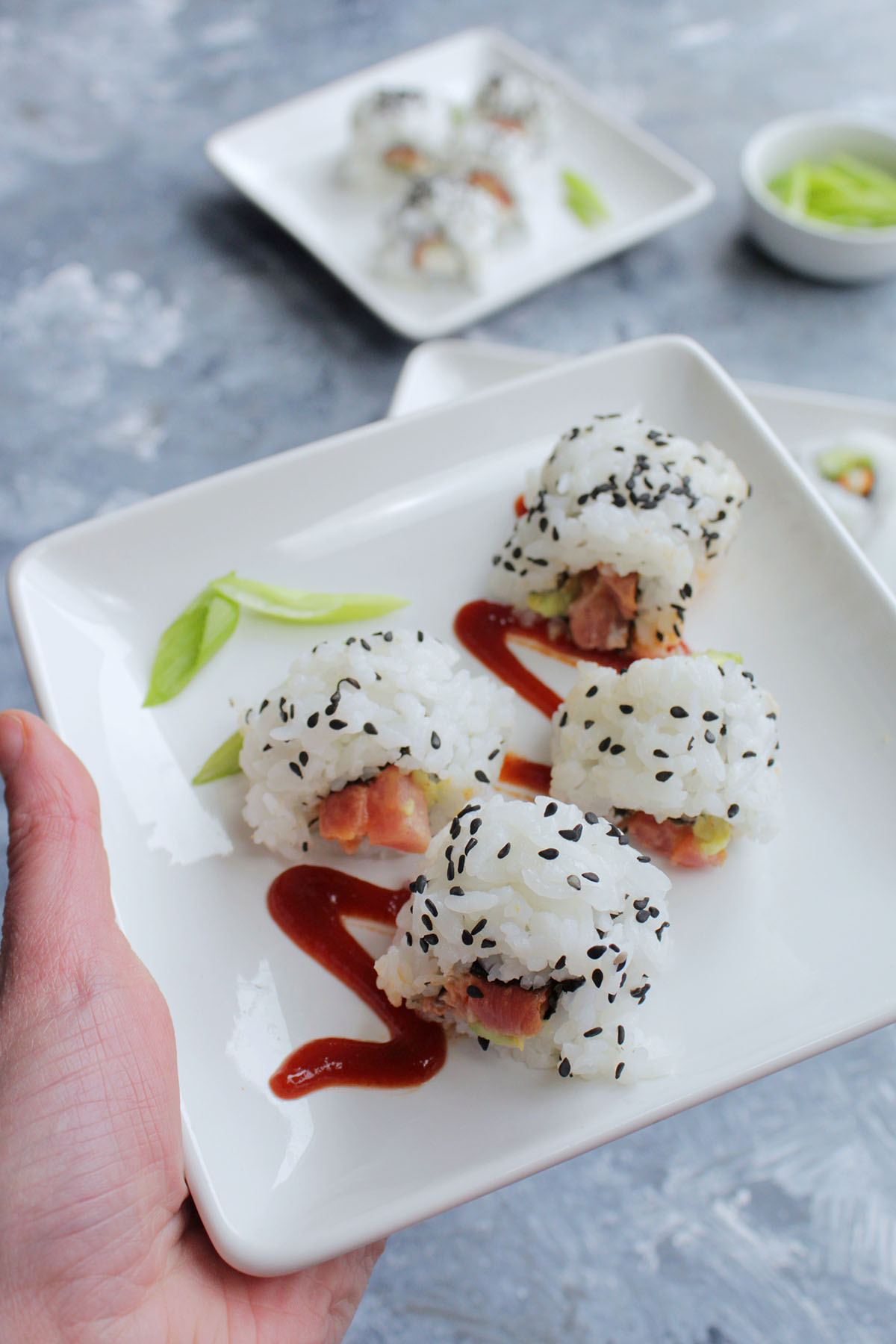In this detailed close-up image, a hand holds a small, square, white ceramic plate featuring an artful arrangement of four sushi rolls. The sushi, wrapped in white rice and sprinkled with dark sesame seeds, showcases a reddish-pink fish, likely tuna, at its center. A squiggly drizzle of red sauce decorates the plate beneath the sushi, adding flair to the presentation. A small green leaf garnish is placed delicately in one corner of the plate. The foreground of the image is crisp and focused, highlighting the details of the hand and the sushi plate. In contrast, the background is slightly blurry but reveals a light bluish table with additional plates of sushi, including another square plate and possibly an oval or rectangular one. There is also a shallow round bowl that seems to contain some kind of green vegetable or garnish, though its exact nature is obscured by the blur.